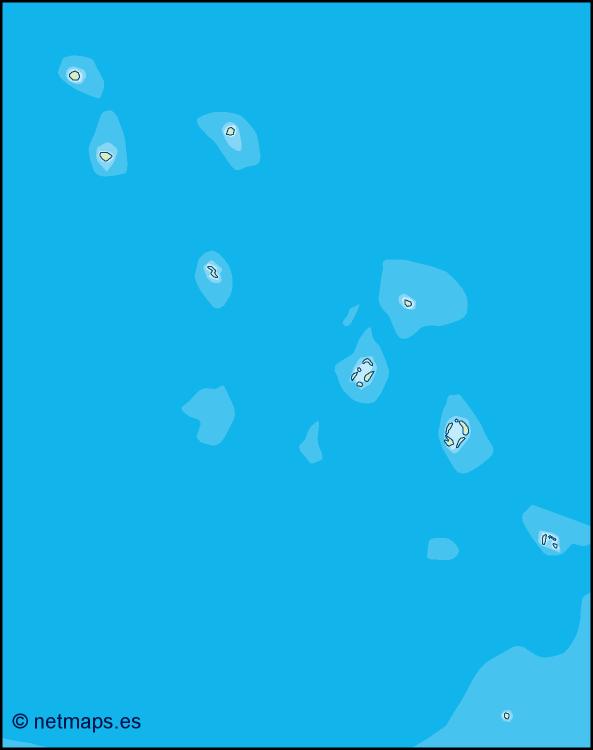The image is a cartoon-style depiction of an archipelago situated in a blue ocean. The map, oriented as a vertical rectangle, shows a series of small, scattered islands depicted in a beige or light tan color, resembling an aerial radar map. The islands appear as tiny shapes in a marine blue sea, with nine primary landmasses angled downward to the right and an additional small island in the bottom right corner. Surrounding these islands are areas of lighter blue, indicative of shallower waters or shorelines. The map is enclosed by a thin black outline, and in the bottom left corner, there is a black or dark blue text reading "Copyright netmaps.es." This plain map provides a simplified, yet detailed representation of the islands within this specific body of water.